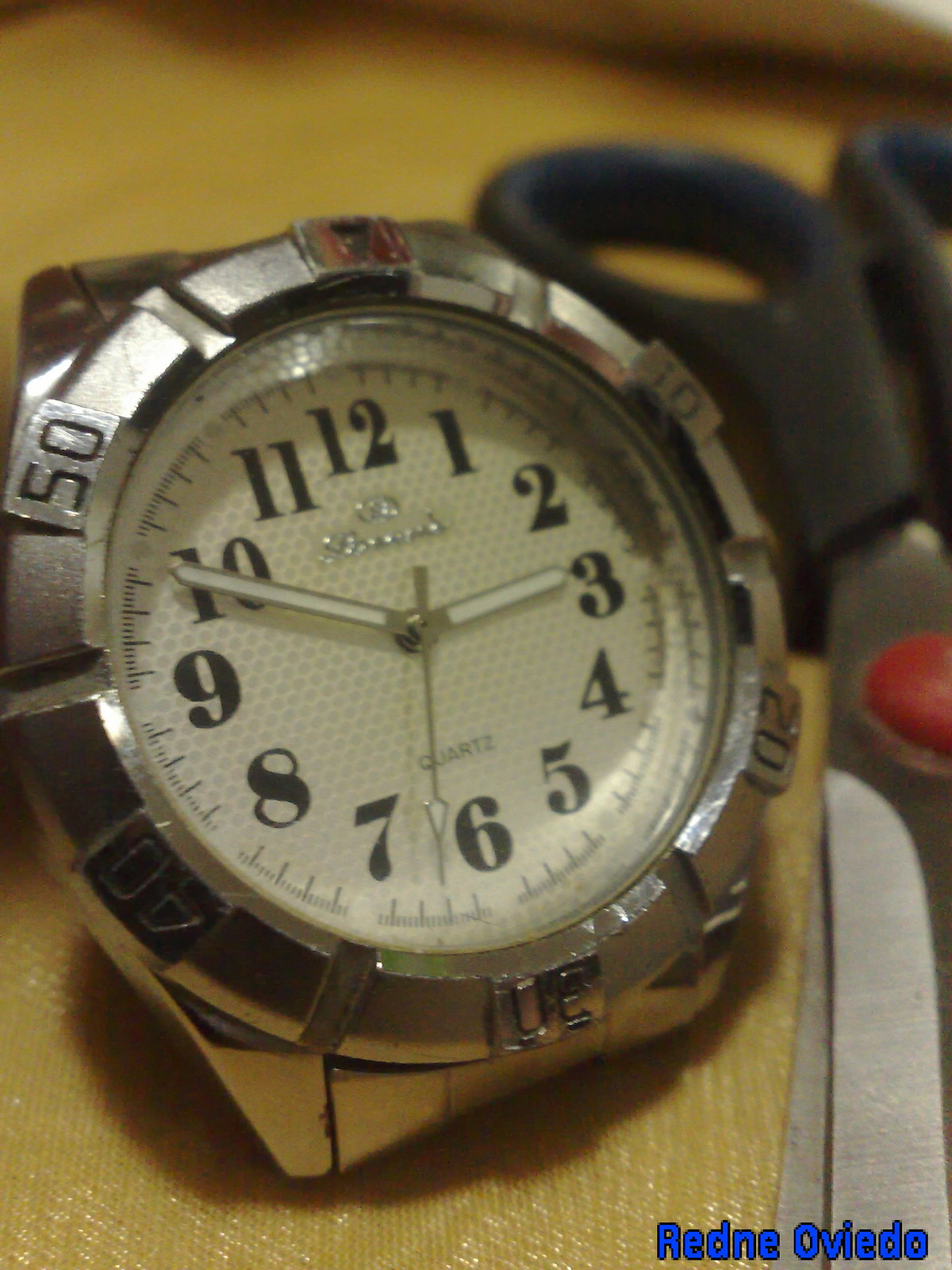In this image, an old wristwatch is prominently displayed on a golden-colored surface. Next to the watch lies a pair of scissors featuring sleek black handles. The watch's face is a pristine white with clear black numerals and elegant white hands. The time shown on the watch is 2:50, with the second hand positioned between the numbers six and seven. Below the hands, the label "QUARTZ" is inscribed in bold, dark capital letters. The watch's exterior casing is metallic and features numerical markers at intervals of 10, 20, 30, 40, and 50. The watch band is also made of metal, matching the casing's finish. In the lower right corner of the photograph, the words "Redne Ovejdo" are written in bright blue letters, adding a pop of color to the scene.